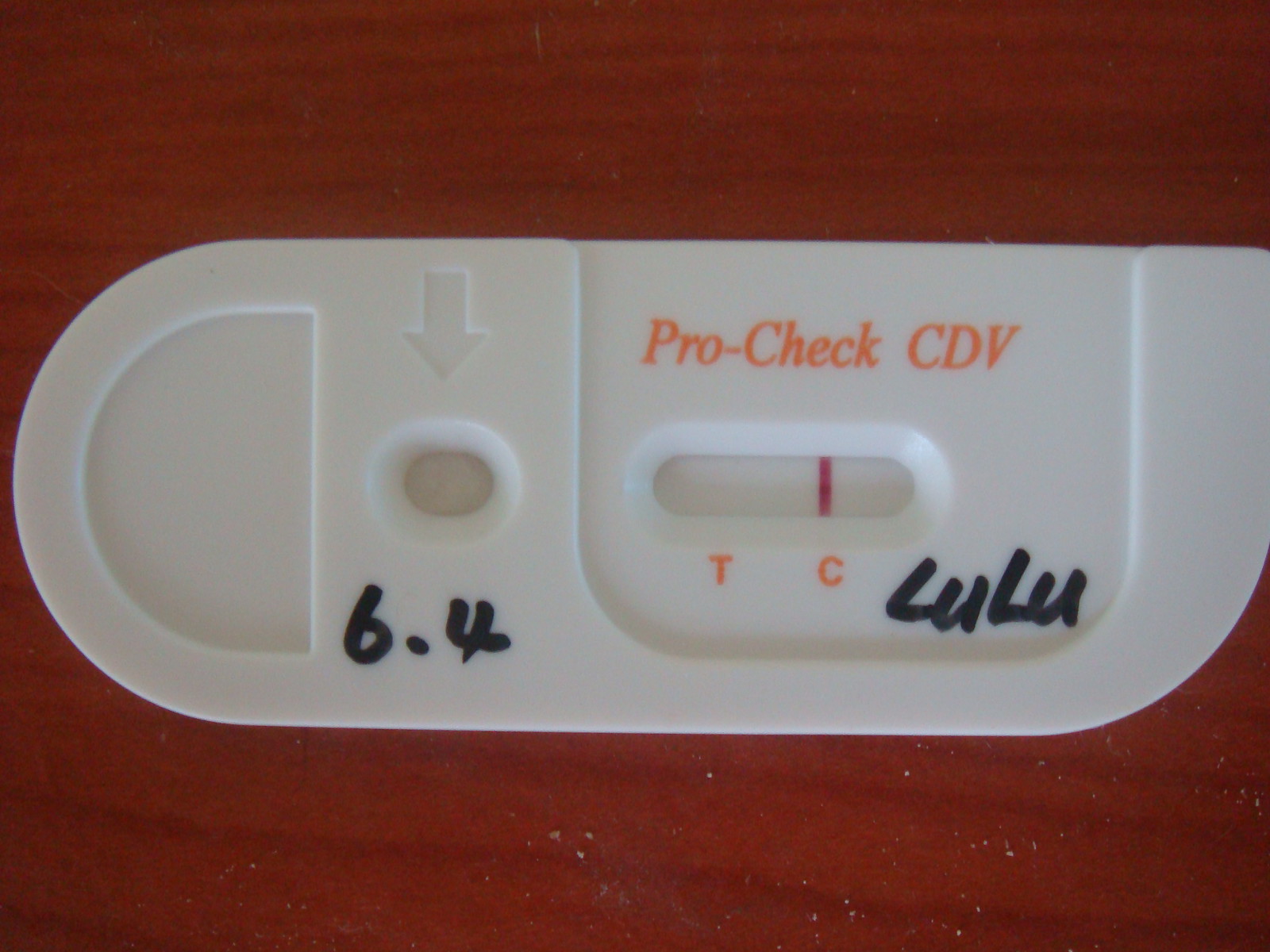This photograph features a COVID-19 self-test kit lying on a table. The test kit is a white plastic device marked with handwritten notes in magic marker, which include the numbers "6.4" and the name "Lulu." The device itself is labeled with "ProCheck CDV" in orange letters, along with the letters "T" and "C." The "C" likely stands for the control line, which is indicated by a visible vertical red line above the letter. An arrow points towards an oval-shaped area where the test liquid is applied. Notably, there is no red line above the "T," suggesting a negative test result. The overall arrangement and markings indicate a COVID-19 screening test.